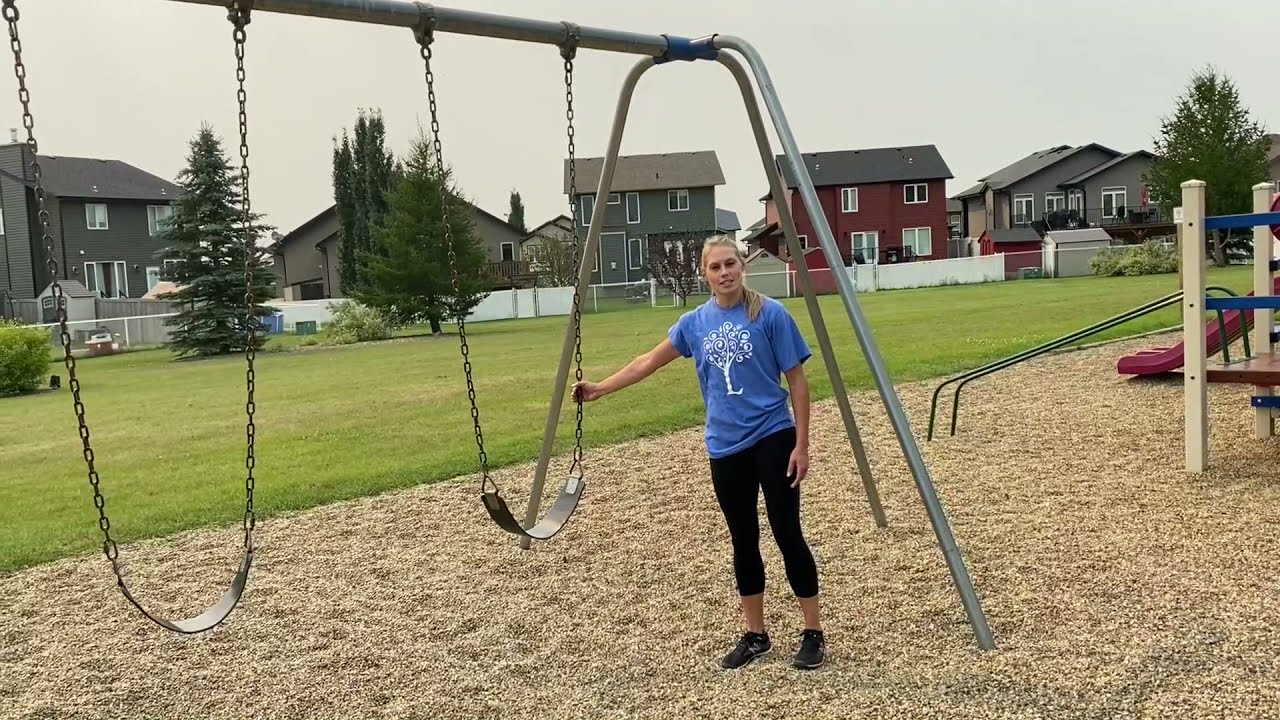This detailed image captures a young Caucasian woman in her 20s, standing next to a swing set at a children's playground in a suburban park. She has long blonde hair tied back in a ponytail, and she is holding one of the chains of the swing with her right hand. The woman is dressed in a blue t-shirt featuring a white letter "L" and black capri yoga pants, complemented by black Nike athletic shoes. She stands on mulch, indicative of a children's play area, with her arm extended to touch the swing. In the background, there is a red slide, various climbing bars, and other playground equipment. Behind the playground, a lush, green lawn and a tall fence delineate the park from the adjacent suburban neighborhood, which consists of closely situated houses in varying colors such as red, blue, and gray. The setting also features scattered tall trees and an overcast, hazy sky, which adds a serene, muted ambience to the scene.